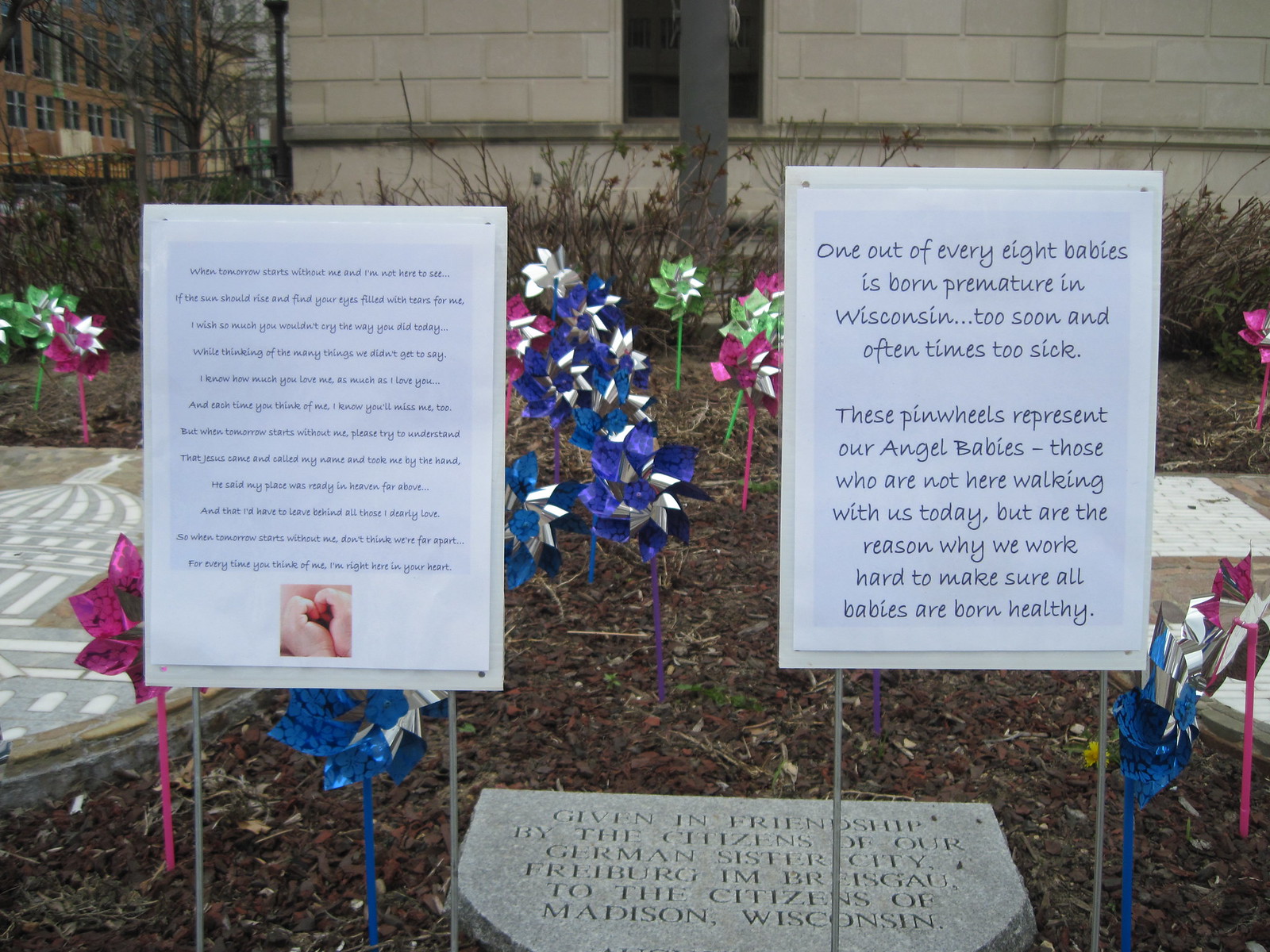The image depicts a somber yet heartfelt scene in an area that resembles a cemetery or memorial. The focal point is a mulched ground adorned with colorful pinwheels—predominantly blue and silver, green and silver, pink and silver, with a few purple and silver ones. These pinwheels are scattered around, each representing a vulnerable "angel baby" who was born prematurely in Wisconsin. 

In the foreground, a grey stone marker lies flat on the ground with the inscription, "Given in friendship by the citizens of our German sister city to the citizens of Madison, Wisconsin." This is surrounded by two vertical signs with grey poles. The sign on the right, easily readable, shares a poignant message: "One out of every eight babies is born premature in Wisconsin. Too soon and oftentimes too sick. These pinwheels represent our angel babies, those who are not here walking with us today, but are the reason why we work hard to make sure all babies are born healthy." The sign on the left is smaller, less legible, but features an image of hands forming a heart shape.

In the background, various buildings frame the memorial area. A white brick building with a fence and pole in front of it is visible directly behind, while another brown building with many windows, possibly a school or apartment complex, is situated in the upper left-hand corner. The landscape is devoid of much grass but features some bushes and weeds, further enhancing the solemnity of this touching tribute to those lost too soon.